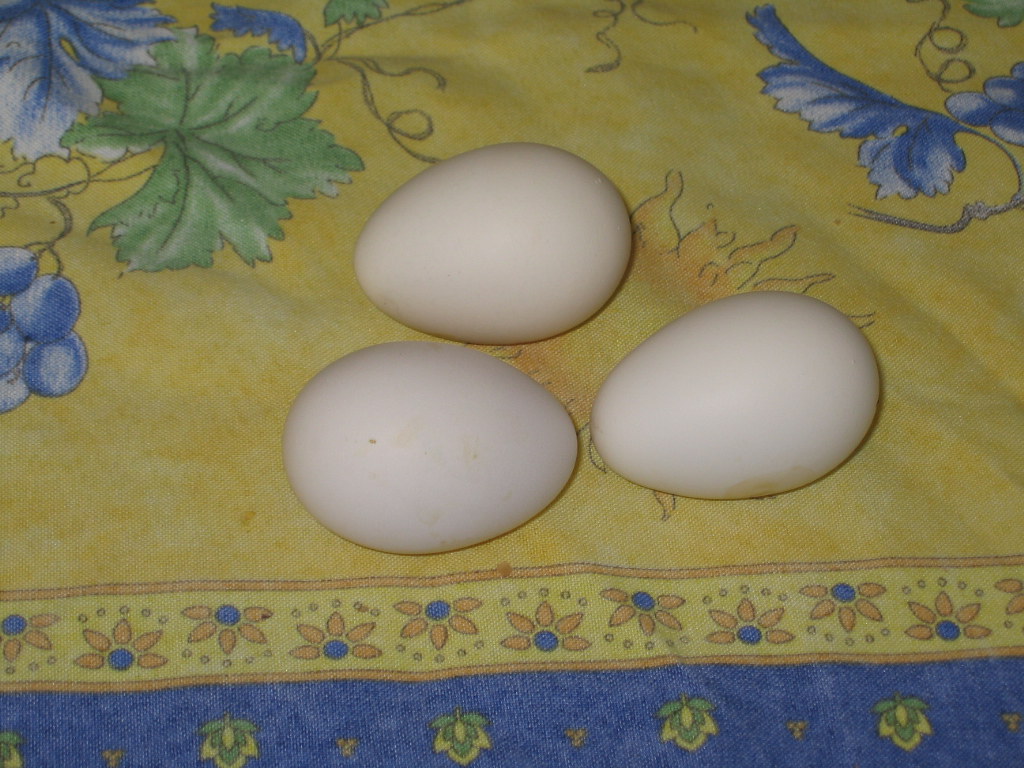This vibrant color photograph features three slightly off-white, naturally appearing eggs, prominently placed on a pale yellow fabric, possibly a tablecloth or placemat. The eggs are arranged in a triangular cluster with two at the bottom and one perched atop, their narrow ends oriented in alternating directions. A noticeable yellow discoloration and a couple of specks can be seen on the rightmost egg. The fabric beneath them displays intricate patterns: blue and white flowers, green leaves, and yellow foliage near the eggs. Surrounding the eggs, there's a delicate border of darker yellow and blue flowers, transitioning to a blue background adorned with green leaves and small orange dots, evoking a sun outline with wisps of orange. This rich tapestry of colors and patterns forms a visually enticing backdrop for the seemingly free-range eggs, almost placing them in the center of a natural, decorative setting.